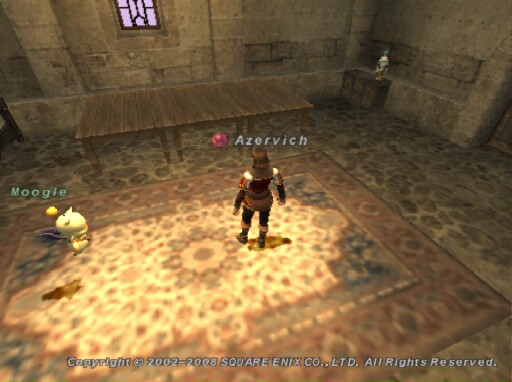This screen capture of gameplay, dating from 2002 to 2008 and copyright Square ENIX Co., LTD, showcases a medieval-looking knight figure. The knight is adorned in dark-colored pants and boots, complemented by a red and gold tunic. With flowing brown hair and the name "AZERVICH" displayed above in a pink bubble outlined in white font, the character stands prominently on an intricately designed area rug featuring shades of tan, brown, blue, white, and gray.

Sharing the rug is a cat-like creature standing upright, identified by the name "MOOGLE" in blue font hovering above its head. The backdrop reveals a stone castle room characterized by a mix of darker and lighter grays. Adding to the medieval ambiance, a wooden table occupies the room, beneath a window that filters in a soft purple light, casting a mystical glow throughout the scene.